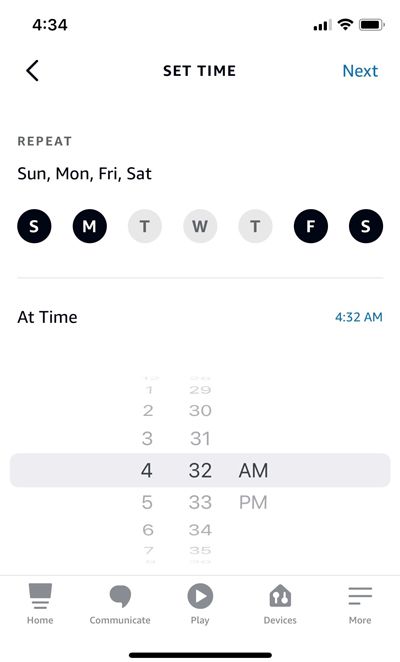The image showcases a cellphone screen displaying an alarm clock reminder interface. In the top left corner, the screen displays the time "4:34." The top right corner features icons for connection, Wi-Fi signal, and battery percentage. Below this, centrally aligned, the interface presents the option to "Set Time" with a "Next" button in blue to its right, accompanied by a left-pointing arrow.

Further down, the "Repeat" section indicates that alarms are set for Sunday, Monday, Friday, and Saturday, visibly highlighted by black circles around the respective day abbreviations. The days that are not selected—Tuesday, Wednesday, and Thursday—are marked with gray triangles.

Underneath this, at the "At Time" section, the time "4:32 AM" is shown to the right, indicating the selected alarm time. At the very bottom of the screen, five icons are displayed from left to right: Home, Communicate, Play, Devices, and More. A black horizontal bar is positioned in the center-right at the bottom of the screen, which features a predominantly white background.